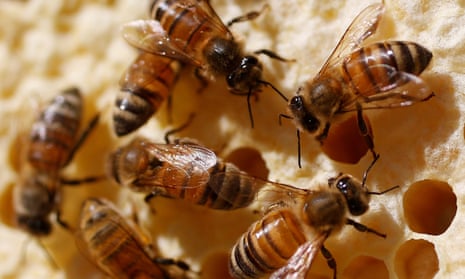This professional close-up photograph showcases a cluster of approximately six to seven honey bees engaged on a honeycomb. The image is triangular in shape, capturing the bees in precise detail. Their bodies display a combination of honey brownish-yellow tones with black horizontal stripes, prominent black heads, long thin legs, and short black antennas. The bees' transparent wings also show a slight brownish tint. The honeycomb they are on is light yellow with visible hexagonal holes, particularly noticeable in the bottom right corner of the image. The focus and lighting in the photograph are exceptionally clear, highlighting even the fine fuzz on the bees. The overall colors in the photograph are predominantly the warm hues of the bees and the honeycomb, with no additional animals, insects, or text present, emphasizing the professional quality and detailed nature of the scene.